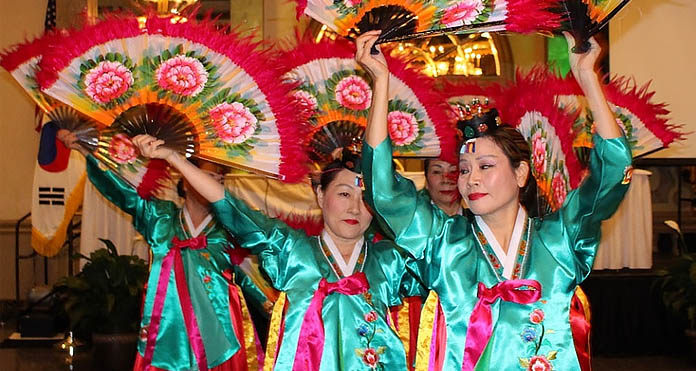The photograph features four Asian women, likely in their 40s or 50s, dressed in brightly colored, shiny satin gowns. Their light green dresses are adorned with pink bows and elaborate floral embroidery in various colors. Each woman is holding a large traditional fan above her head. These fans are decorated with three flowers, in shades of pink, green, white, and yellow, and edged with vibrant red.

The background reveals a setting that suggests a formal or religious ceremony. There's a mix of elements including a white-and-brown wall, possibly a cloth or table, and some plants. To the left, part of what appears to be a Korean flag is visible, and light shines through what looks like stained glass between the women's raised arms. Additionally, details of a stage with a white curtain and wooden elements can be seen, along with a railing that might lead up to the stage. All the women have black hair and are wearing red lipstick, enhancing the vividness of the scene. The overall color palette of the image includes pink, white, green, yellow, orange, brown, off-white, red, and blue tones.